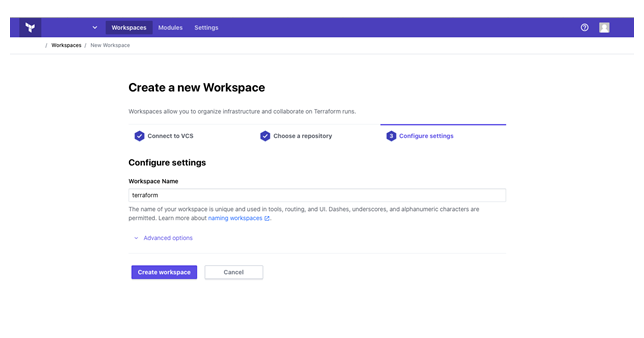The image features a user interface for creating a new workspace on a platform. The top of the UI has a blue background with several sections. On the left side, there's a darker blue square with a symbol resembling a distorted triangle or a "T." Adjacent to it is a plain blue square followed by a darker blue square that has the white text "Workspaces". Next to this is a blue square with two sections labeled "Modules" and "Settings". On the right side, there's a circle with a question mark and an empty profile picture.

Below this, against a white background, the black text reads "Workspaces" with "New Workspace" written in gray to its side. At the center, the prominent black text states "Create New Workspace". Below this, in light gray, the text explains that "workspaces allow you to organize infrastructure and collaborate on Terraform runs."

Three blue hexagons with different symbols appear next; the first two have white checkmarks, while the third has the number three inside. 

- The first hexagon says "Connect to VCS" in black.
- The second reads "Choose a Repository".
- The third, highlighted by a blue line above it, states "Configure Settings".

On the left side, under the "Configure Settings" heading, is a text box with "Terraform" entered into it. Guidance in gray text explains that the workspace name is unique and used in tools, routing, and UI, allowing dashes, underscores, and alphanumeric characters. A clickable link in blue text reads "Naming Workspaces."

Underneath this link are the words "Advanced Options" also in blue. At the bottom of the interface, there are two buttons: "Create Workspace" and "Cancel."